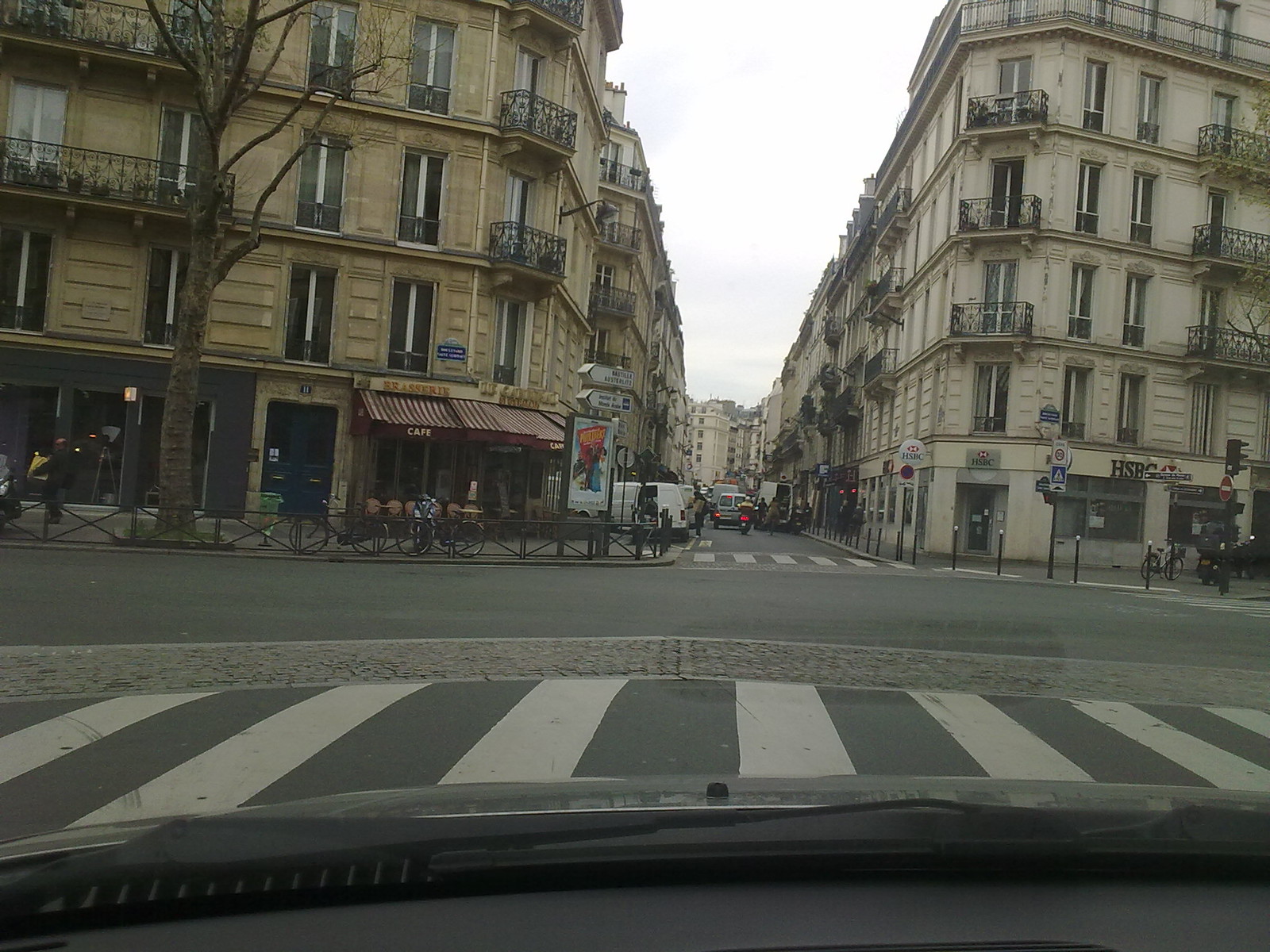The image captures a bustling European downtown street scene, viewed from the inside of a vehicle, likely through its windshield. In the foreground, there is a crosswalk directly in front, beyond which lies a cobblestone sidewalk. The street extends into an alleyway nestled between two ornate four-story buildings with intricate balcony designs, reminiscent of 1800s architecture. The building on the right is marked with an HSBC sign, while those on the left house various shops and cafes, including signs for "Cafe" and "Brasiri." Bicycles and motorcycles are parked along a fence and railings beside the sidewalk. Pedestrians are seen walking, standing, and entering the alleyway or street between the buildings. Vehicles are also present, adding to the dynamic, busy atmosphere. Overhead, the sky is cloudy, emphasizing the typical weather of the scene. The detailed architecture and vibrant street life suggest a charming European city, potentially resembling those found in France.